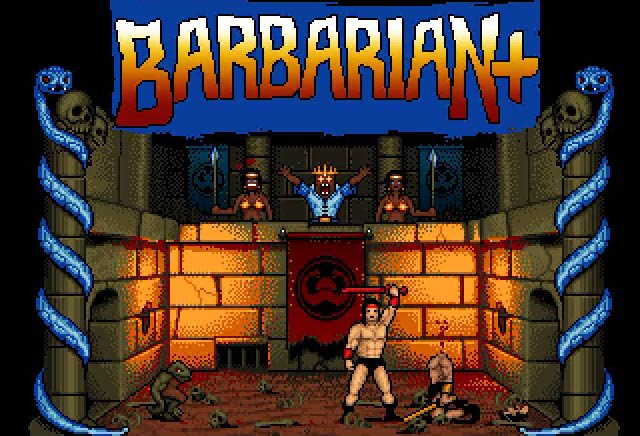The image appears to be a detailed screenshot from an older 8-bit video game called "Barbarian," with the title displayed prominently in white, yellow, and orange text on a blue background at the top. At the bottom right of the title, there is a plus sign. The setting is reminiscent of a medieval castle or warrior's arena, featuring a short wall at the back and on both sides, with poles on each side that have blue snakes climbing up them. Above the wall stand two women in bikinis and a man wearing a blue outfit with his arms raised in a V shape, as if triumphant or celebrating. Below the wall, a man dressed in just black underwear holds a red shawl. Another character, wearing armbands, boots, and shorts, is in the foreground, seemingly in a combative stance, possibly holding a red sword, suggesting a dueling or battling scenario. The image's dark tones and colors, along with the pixelated graphics, evoke the nostalgic feel of vintage video games from the Nintendo era.